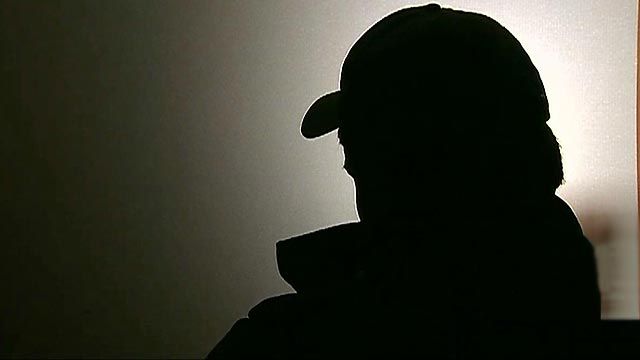The image captures a striking silhouette of an older man wearing a hat and a jacket with a distinct collar, set against a gradient background that transitions smoothly from white on the right to black on the left. Seated in the darkness or in front of a light source, only the man's silhouette is visible from the chest up, leaving his facial features and attire obscured. The focus is solely on his shadowy figure, evoking a sense of mystery as to why he remains hidden in the shadows.